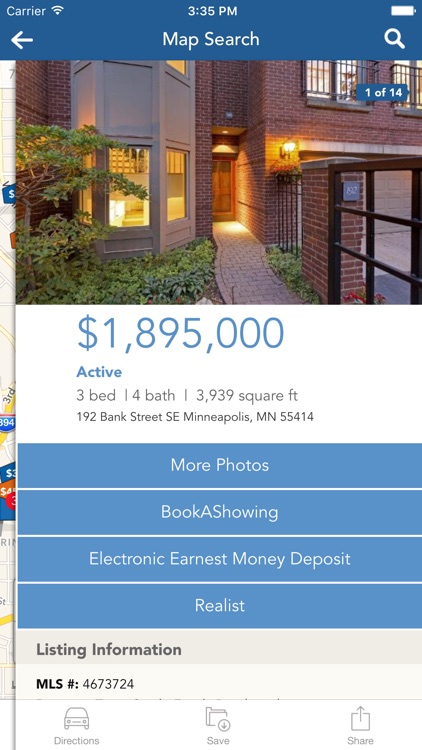Here is a detailed version of the caption:

The image is a screenshot of a property listing search displayed on a smartphone. The listing is for a brick house located at 192 Bank Street, Southeast, Minneapolis, Minnesota, 55414. The house is currently active in the market, listed at a price of $1,895,000. The property features three bedrooms, four bathrooms, and has a total area of 3,939 square feet.

The visual portion includes a clear picture of the front facade of the brick house, showing the walkway leading up to the front door, surrounded by windows and a small fence on the right side. There is also some greenery visible on the left side of the walkway, adding to the home’s curb appeal.

Additional options under the listing allow the viewer to request more photos, book a showing, make an electronic earnest money deposit, and view the listing information along with the MLS number 4673724. There are also options to get directions to the property, save the listing, or share it.